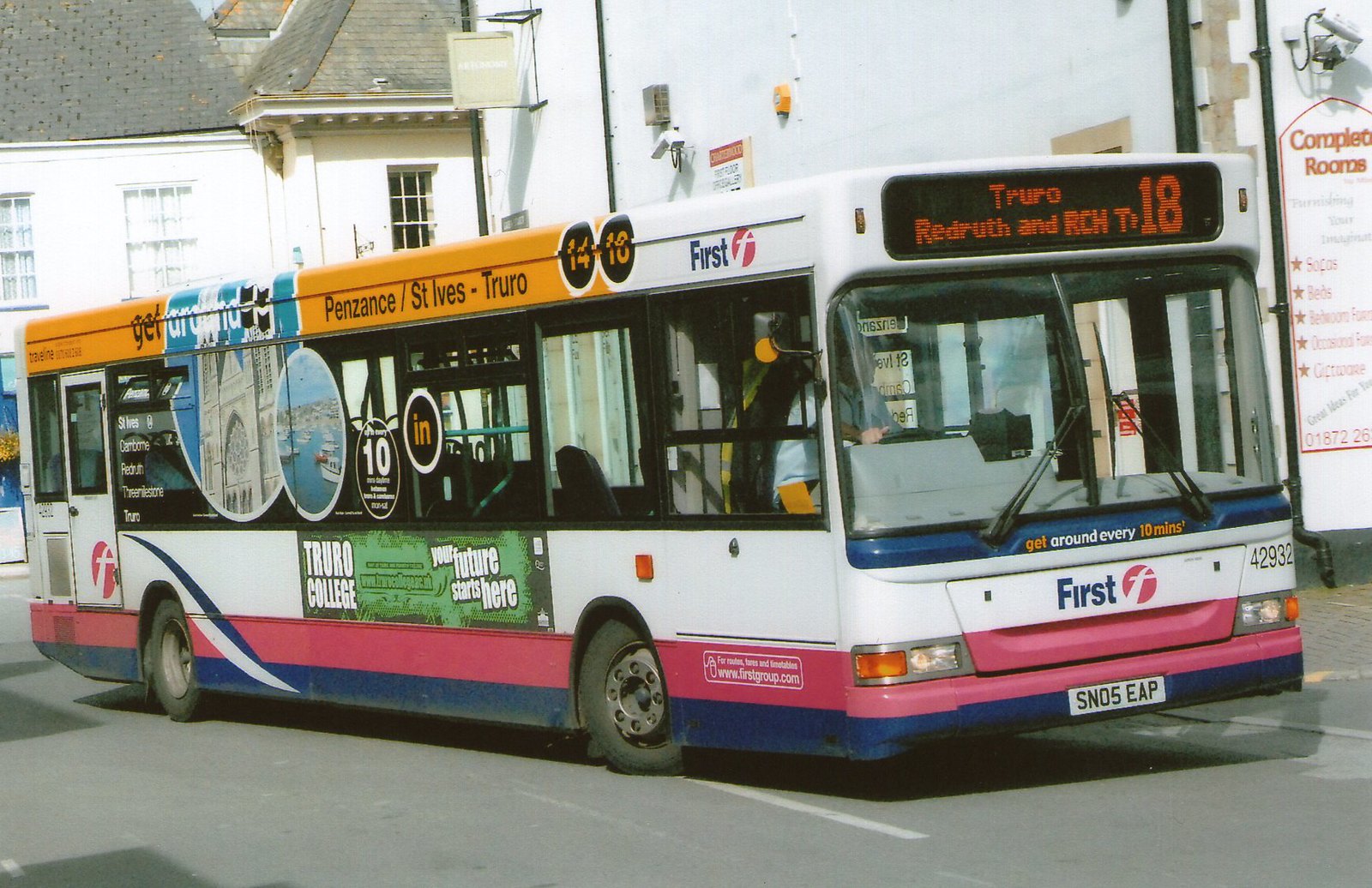The photograph captures a city bus positioned at an angle where the front is facing the right and the rear is off to the left. Prominently displayed above the windshield, the destination sign reads "Truro" with additional text "Redruth RCH2" and the bus route number "18." The bus, primarily white, features an orange stripe at the top with black lettering indicating its route: "Penzance / St. Ives - Truro." The side of the bus displays various advertisements, including one for Truro College with the slogan "Your future starts here." Although the bus appears parked in a city with surrounding buildings, there is no visible sign of passengers, aside from the bus driver seated at the front. The front of the bus also showcases the word "First" in dark blue, complemented by pink accents and a dark blue border along the bottom.